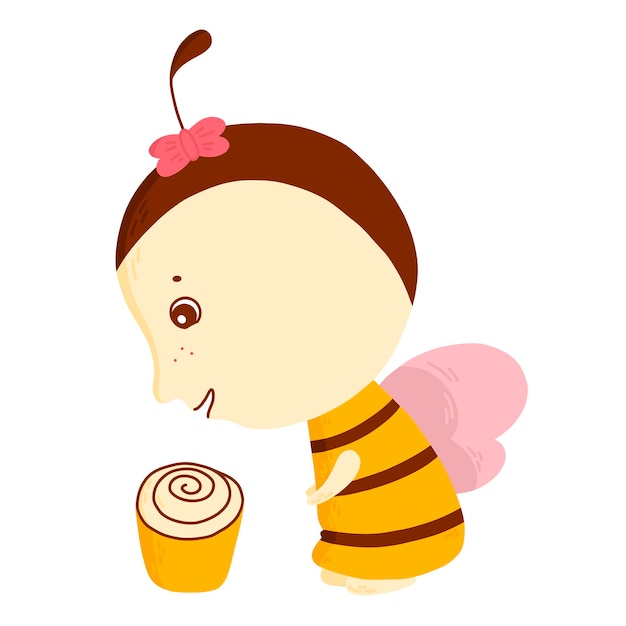In this image, we have a detailed cartoon illustration of a little girl dressed as a bumblebee. She has a large, round face painted a creamy flesh color, with slightly darker shading down the bridge of her nose for depth. Her prominent brown eyes are round and accented by a few freckles beneath them, and she wears a cheerful, open-mouthed smile. Her dark brown hair encircles her head and is adorned with a pink bow shaped like a butterfly, from which a brown antenna protrudes. 

Her body is oval-shaped and predominantly dark yellow with brown stripes, resembling a bee's body, and she has delicate pink wings on her back. The girl is depicted in a side view, standing and gazing down at a small cartoon cupcake on the ground. The cupcake features white swirly frosting and a dark yellow base. The entire scene is set against a clean white background, emphasizing the delightful and whimsical nature of the illustration.